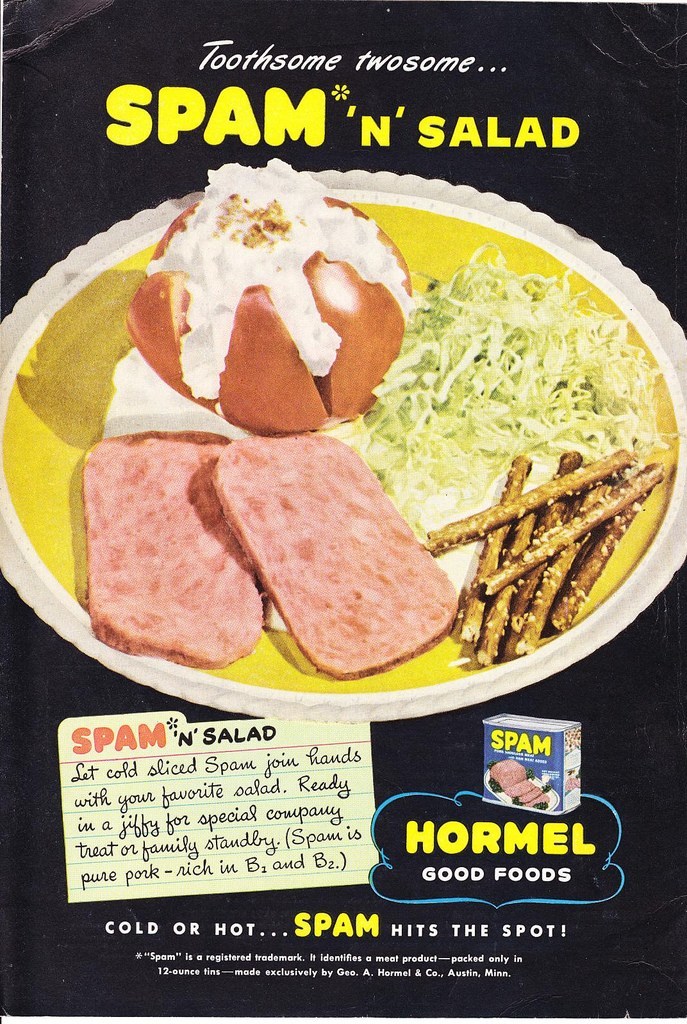This is a vintage advertisement from Hormel Foods promoting the versatility of Spam. Centered in the image is a photograph of a paper plate containing an assortment of food items. Arranged on the plate, starting from the bottom, there are two slices of Spam, some chopped lettuce, a few pretzel sticks, and a round dessert resembling a bun delicately sliced into six sections, filled with white cream, forming a flower-like shape. At the top of the advertisement, the text reads "Toothsome twosome... Spam and Salad" in white and yellow fonts. Near the bottom, a small card reiterates, "Spam and Salad. Let cold sliced Spam join hands with your favorite salad." The accompanying description highlights Spam's appeal as a convenient, nutritious product rich in B1 and B2 vitamins, made exclusively in 12-ounce tins by G.O.A. Hormel Co. in Minnesota, emphasizing its suitability for both special occasions and everyday meals.